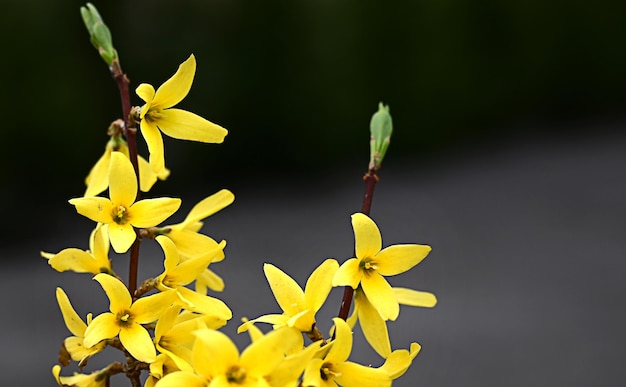This image depicts a close-up photograph of vibrant yellow flowers against a blurred black and gray background. The focus is on two vertical stems on the left side of the image, each adorned with several small flowers. Each flower consists of four elongated, skinny petals that are a vivid yellow, contrasting sharply with the dark background. The center of each flower is a darker, reddish-brown color. At the top of each stem is a green bud that hasn't yet blossomed, providing a touch of verdant green to the overall composition. The stems appear dark reddish-brown in color. The image is closely cropped, showing only the top part of the flowers and not extending to the middle or lower parts. The stark contrast between the bright yellow petals and the dark background emphasizes the flowers' vibrant and visually appealing nature.